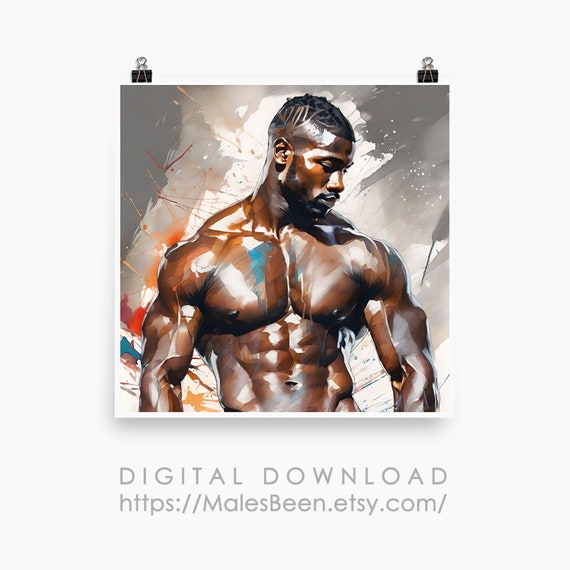This image features a stylized, digitally enhanced portrait of an exceptionally fit African American man, resembling a bodybuilder, depicted from the waist up. The figure, a handsome young man in his early 20s with large shoulders, muscular arms, and a washboard stomach, has dark hair styled with a design on the side, and he sports a slight beard and mustache. He is shirtless, bodily facing the camera but looking down and to the right, giving a contemplative expression. The photograph, which seamlessly blends photographic realism with digital artistry, is complemented by vibrant splotches of paint in hues of white, blue, red, and orange. These splashes extend across the man's torso and the predominantly gray background, creating a dynamic and powerful visual effect. The image is vertically rectangular with a faint light gray border, and it is secured by two binder clips at the top corners. At the bottom, an advertisement in gray text reads, "Digital download," followed by the URL "https://malesbin.etsy.com."